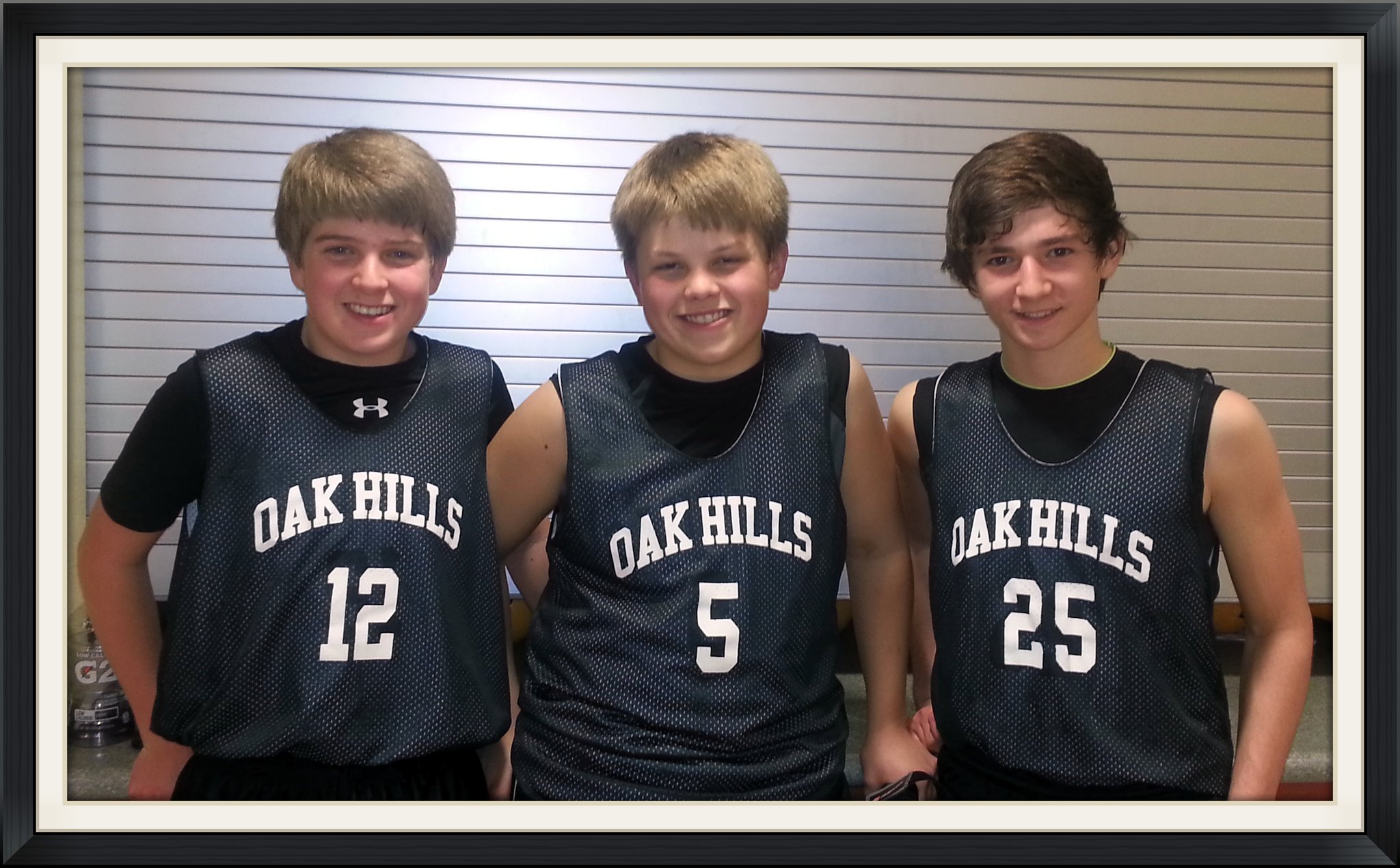In this image, three boys are posed in front of a background made up of horizontal thin white slats, which could be a metal or overhead door, possibly from a canteen or a closed cafeteria window. The boys, appearing to be between 12 to 14 years old, are dressed as basketball players. They are all smiling and sporting Oak Hills jerseys with white text; the jerseys appear to be dark green and made of a mesh material that is slightly transparent. The boy on the left, wearing jersey number 12, has a black short-sleeved undershirt featuring what looks like an 'H' at the neckline, possibly a Hurley or Under Armour logo. The boy in the middle, sporting jersey number 5, and the boy on the right, in jersey number 25, both have black sleeveless undershirts. Their hair is relatively short, with the boy on the right having medium brown hair and the other two boys sporting lighter brown or dark blonde hair. There is a G2 Gatorade bottle visible on a counter to the left of the photo. The entire image is framed with a white outline and an additional black border.